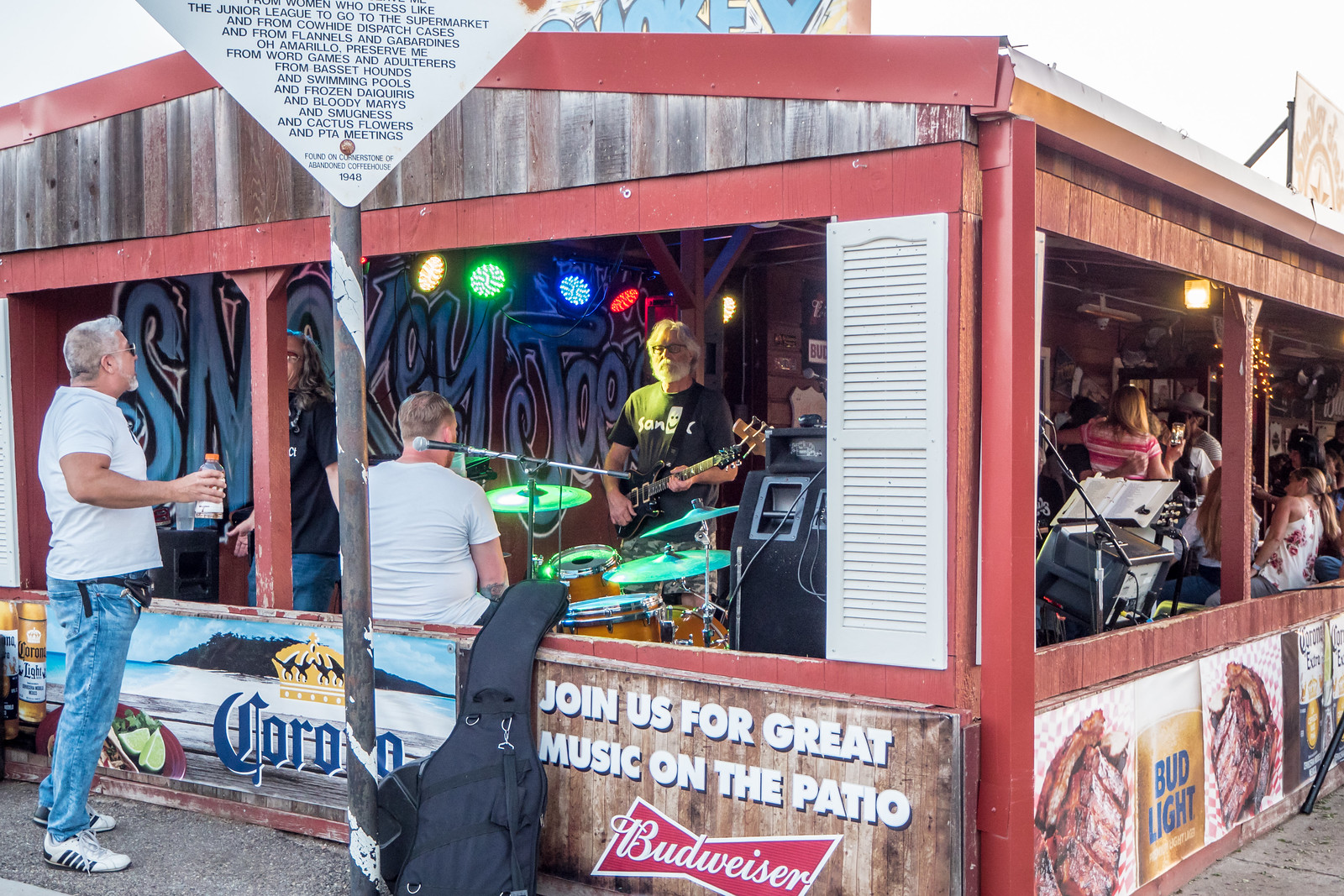The image depicts a lively scene at an open-air structure, which serves as a combination restaurant and patio bar. The structure has a roof with large, open windows, allowing a view both inside and out. Inside, a band is performing; prominently featured are a guitarist in a black T-shirt and a drummer in a white T-shirt with brown hair. The guitarist stands center-stage, while the drummer sits at his drum set. 

Adjacent to the band, on the right side of the image, some patrons are seated and standing, attentively listening to the music. Multicolored lights enhance the ambiance inside, and the brown wooden structure is outlined in red, giving it a warm and inviting look. One man, dressed casually in a white T-shirt, blue jeans, and Adidas shoes, stands outside the structure, holding a plastic bottle, possibly Gatorade, and watches the band through the open windows.

The outside walls of the structure are adorned with a colorful mural and several advertisements, including ones for Corona, Budweiser, and Bud Light, indicating the availability of these beverages. Above the structure, a prominent, quirky sign catches the eye, reading: "The Junior League to go to the supermarket...from flannels and garbrandines, oh Amarillo, preserve me from word games and adulterers, from basset hounds and swimming pools, and frozen daiquiris and Bloody Marys and smugness and cactus flowers and PTA meetings." This intriguing message adds a layer of character to the eclectic ambiance of this rural American venue from an abandoned coffee house cornerstone dated 1948.